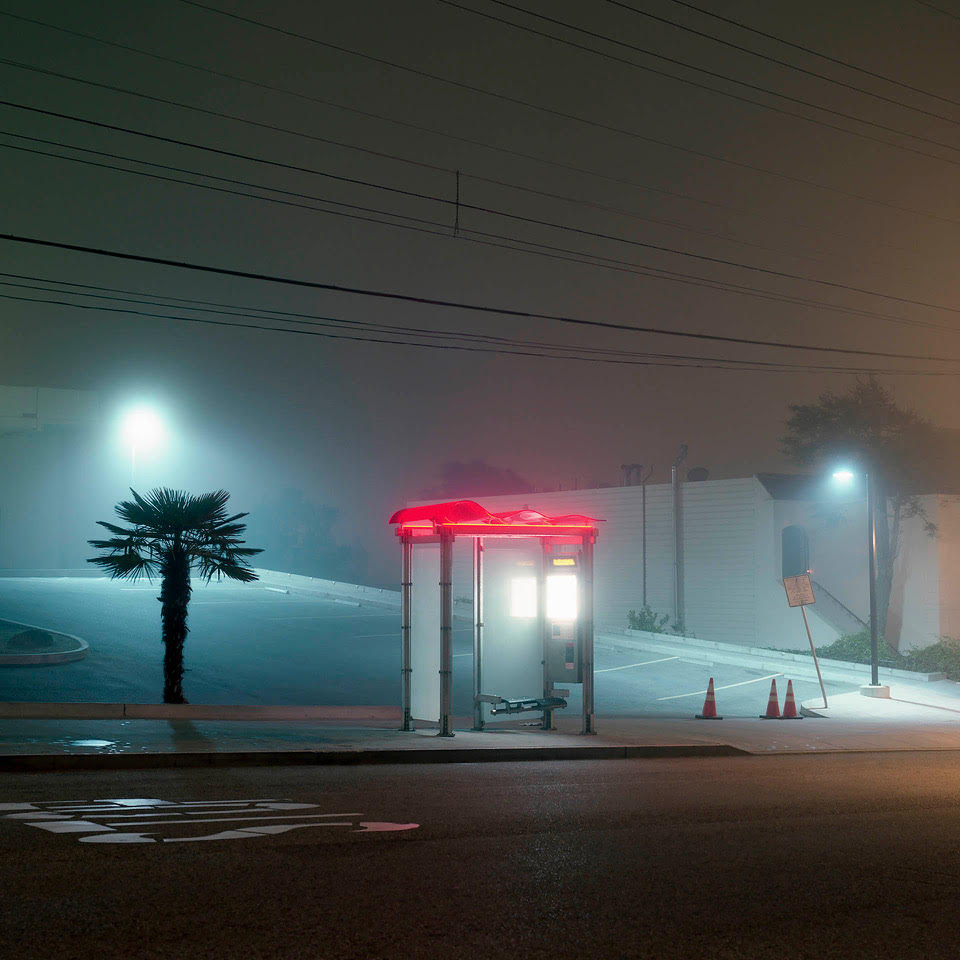The image captures a foggy, misty night scene set outside on a deserted street. The sky is heavily overcast with dark gray clouds. In the foreground, two black power lines stretch horizontally across the scene. Dominating the middle of the picture is a clear glass bus stop structure with a red roof that emits a warm glow. Inside the bus stop, metal prongs can be seen, which might be small seats or supports. A white light illuminates the interior of the bus stop.

To the right of the bus stop, three traffic cones are visible along with a road sign that appears to be crooked, possibly from being hit. Nearby, a short palm tree approximately the same height as the bus stop stands out on the left, highlighting the otherwise stark surroundings.

The street in front of the bus stop is empty, its asphalt surface appearing wet or glossy from the fog, with the word "STOP" painted in white. A deserted parking lot lies behind the bus stop, marked with white parking spaces. Two streetlights are present in the image, one closer to the foreground on the left and another further in the background within the parking lot, both casting a diffused glow partially muted by the fog. A small white building and a sidewalk are also visible further in the distance, partially obscured by the mist.